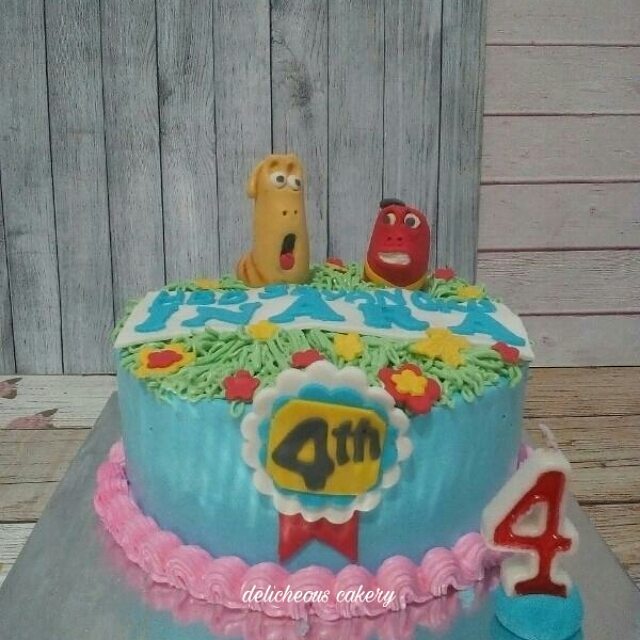This photograph captures a detailed and vibrant birthday cake set on a backdrop of slatted wood panels, featuring gray vertical slats behind and beige horizontal slats to the side. The cake, designed to celebrate a fourth birthday, is anchored on a silver board and bordered with extensive, thick pink-swirled frosting. 

At the center is a blue ribbon medallion with decorative floral patterns, inscribed with "Fourth" on a yellow field. Draped below it are red ribbon details, enhancing the celebratory theme. The cake's base is wrapped in bright blue frosting.

Prominently atop the cake is a lush, green stringy grass icing, adorned with colorful flowers and small birds. Two cartoon characters emerge from the icing: a vertically elongated, beige dog-like figure with bulging eyes and an open mouth on the left, and a smaller, red character with a similarly startled expression on the right.

Inscribed on the cake in blue, a white banner reads "HBD Enara," though some of the text is partially obscured. Nearby, a candle shaped like the number four stands on a bright blue marshmallow next to the cake, yet to be lit.

Completing the cake's presentation, an overlay text at the bottom reads "Delicious Cakery," spelled uniquely as "D-E-L-I-C-H-E-O-U-S C-A-K-E-R-Y." This joyful and detailed cake sets the perfect scene for a memorable fourth birthday celebration.